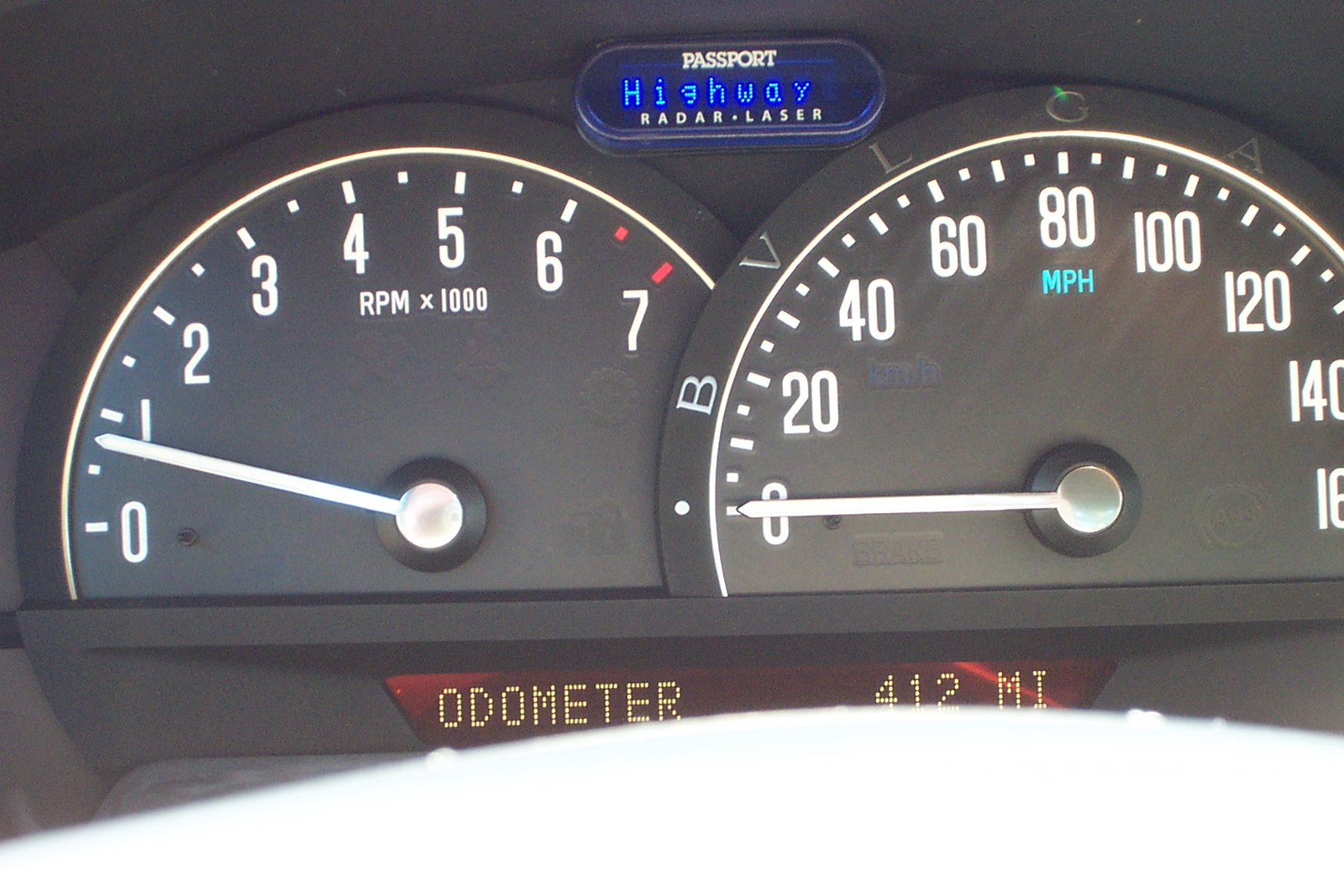In this photograph, we see the dashboard of a car, predominantly black, set against a dark background. At the top of the dashboard display, the text reads "Passport Highway Radar • Laser," presumably indicating a radar detector device. The odometer at the bottom shows a reading of 412 miles. On the right side of the dashboard, the speedometer is displayed, which measures speed in miles per hour (MPH) and currently points at zero. The speedometer scale ranges from 0 to 180 MPH, with the letters "BVLGA" surrounding it. On the left side, the tachometer, which measures engine revolutions per minute (RPM), is slightly above the halfway mark but below the number 1, suggesting it is between 500 and 1000 RPM. The tachometer scale ranges from 0 to 7, and just below the numbers, it says "RPM x 1000."